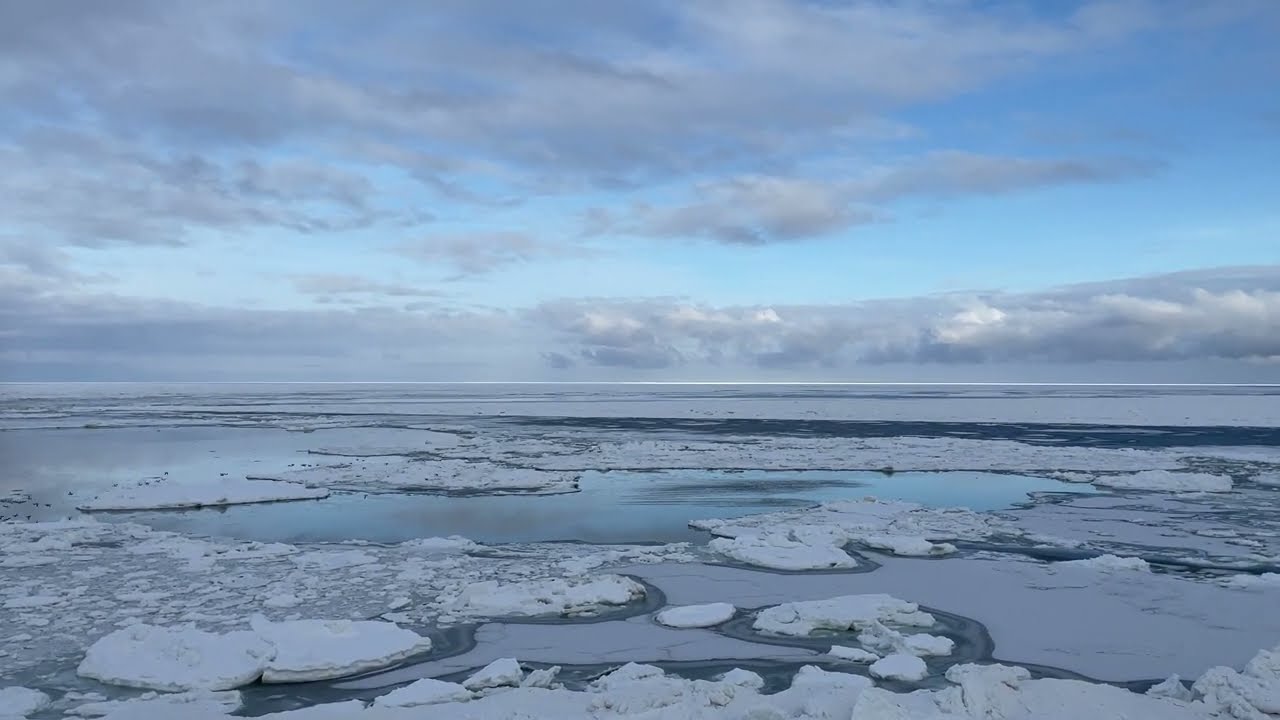The photograph captures a vast salt lake, partially frozen under winter's grasp. The bottom half of the image reveals the lake's surface dotted with jagged breaks in the ice, exposing pools of water lightly frosted but not solid. Deposits of salt mark the landscape where the water has receded, leaving behind intricate formations that resemble clumps or even rocks. A distinctive blue border outlines these salt deposits, hinting at variations in density or texture. Horizontally bisecting the photo, the horizon appears as a fine white line demarcating the lake from the sky. Above, a low layer of dark clouds looms, mingling with patches of blue sky and a few incoming dark clouds from the upper left corner. Despite the overcast appearance, the scene retains a brightness that contrasts with the cold, barren landscape below. No buildings or people intrude upon this serene, icy panorama, emphasizing the solitude and raw beauty of nature in its winter stillness.